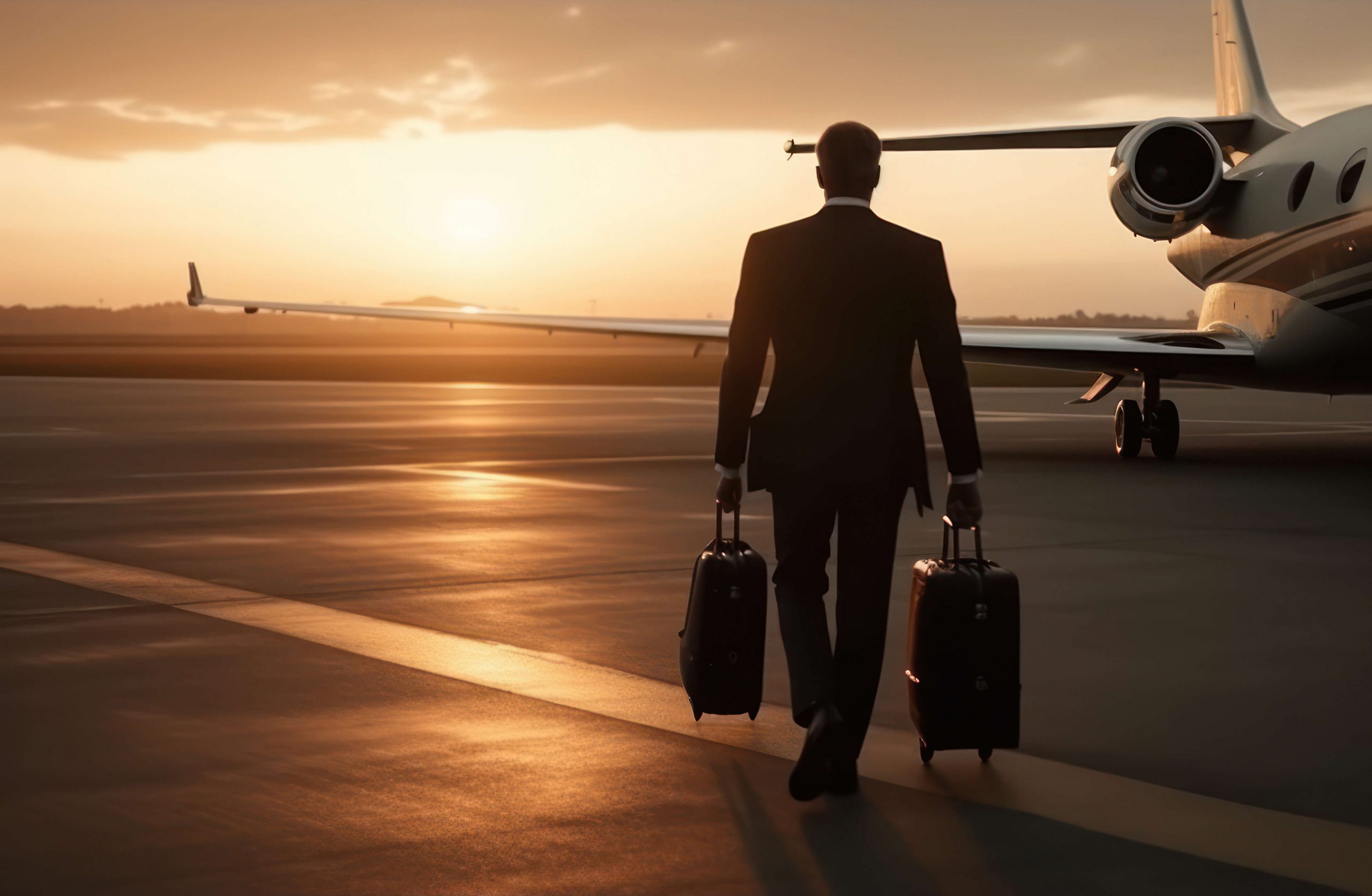In this evocative photograph, a tall gentleman in a black business suit, highlighted by a white shirt with visible cuffs and collar, is seen from behind walking towards a sleek, white private jet with gray accents on an airport tarmac. The man is silhouetted against a captivating sky, aglow with a yellow-golden-orange hue, suggesting the magic hours of either sunrise or sunset. To his right, he rolls a red suitcase with extendable handles, while his left hand carries a shorter, black bag. The tarmac, lined with white markings, reflects the soft sunlight, adding to the serene yet purposeful ambiance of the scene. Far off to the right, the private jet’s engine and wing are easily visible, with the wing stretching almost the entire width of the photograph. The horizon is a flat expanse adorned with low-lying clouds and faint, mountainous terrain, all bathed in the golden light, with bumpy clouds gradually turning gray as they extend to the right, completing this striking and atmospheric composition.